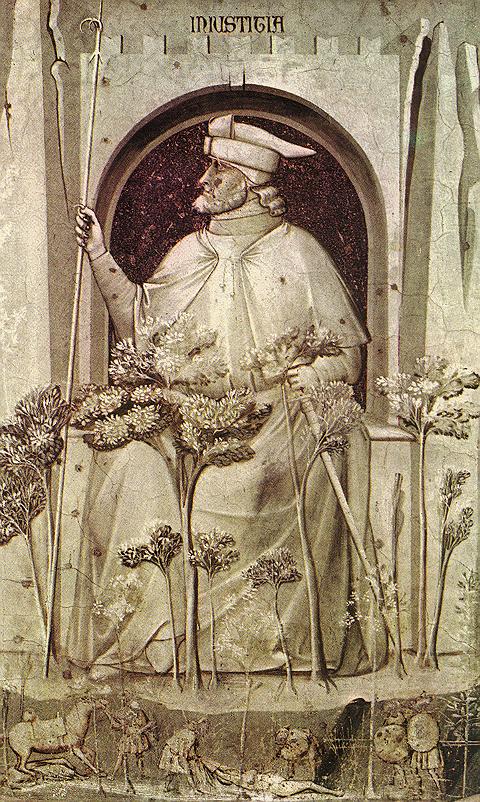This detailed artwork, likely an older print or painting, portrays what appears to be a regal or religious figure seated on a throne with intricate stonework and natural elements. The central figure, possibly a king or a deity, is depicted in great detail. He sits in an arched stone alcove, facing to his right but his body oriented towards the viewer. He holds a long narrow staff with pointed, elongated fingernails on his right hand, while his left hand grasps the hilt of a sword that leans against the ground. He wears a pointed hat extending backward, has long wavy hair down to his neck, a short pointy beard and mustache, and is draped in a robe reminiscent of papal attire. 

In the lower portion of the image, various scenes unfold on what appears to be steps or a mirrored surface. On the left, a man struggles to control a spooked horse, while another man appears to be dragging a lifeless body toward the horse. Two soldiers with large shields and undefined figures or animals add to the complex narrative at the bottom of the picture. Tall and shorter trees rise in front of the central figure, contributing to the multi-layered composition. The artwork employs a color palette of faded olive greens, light browns, and tans, lending it an aged appearance. Above the seated figure, in the archway's upper stonework, are carved letters, which might read "M-I-U-S-T-I-G-I-H" or "I-N-R-I-S-T-I-G-I-A," adding to the enigmatic aura of the piece.